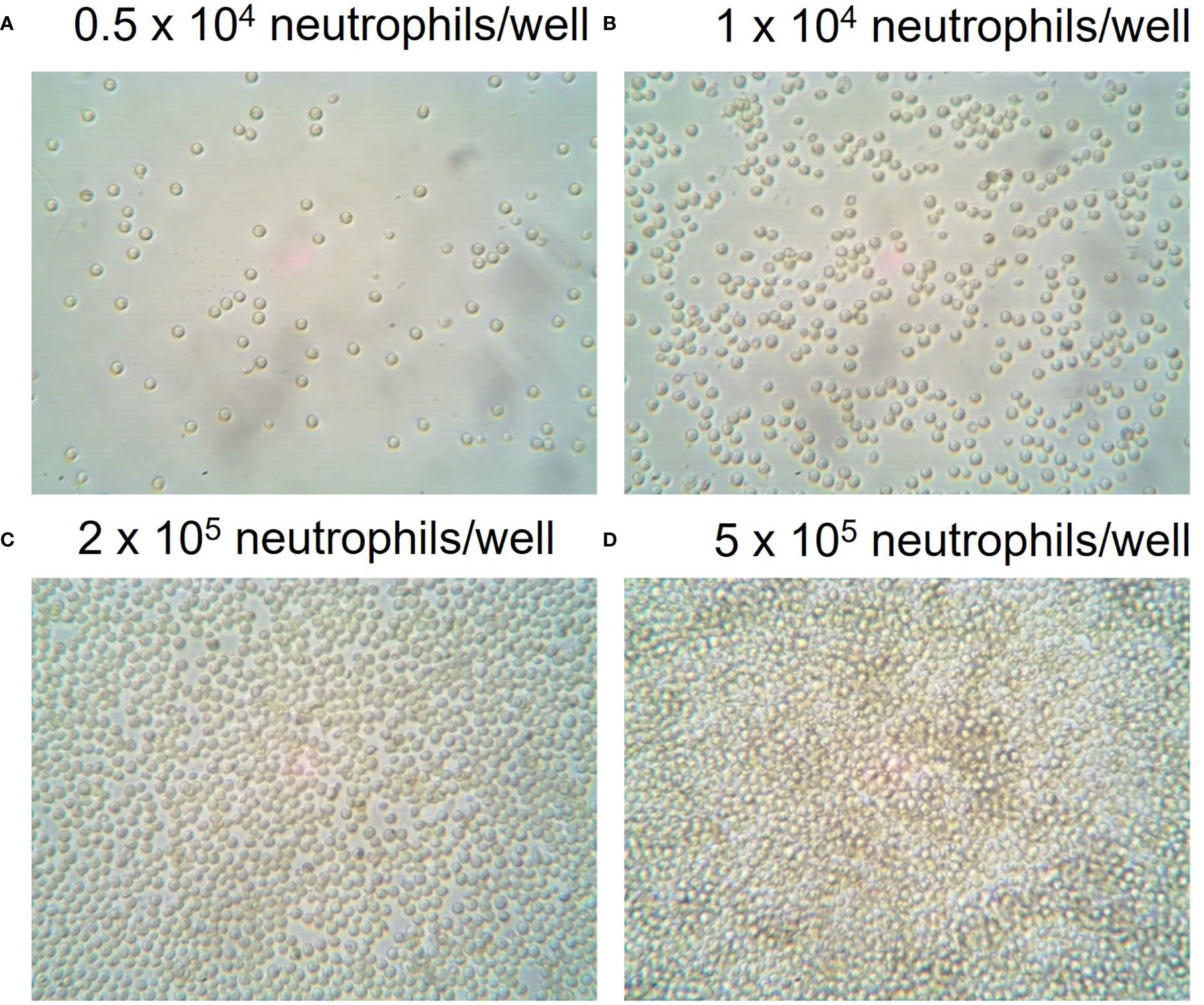The image consists of four detailed, close-up microscopic views labeled A, B, C, and D in black text at the top left corner of each image, depicting an increasing density of neutrophils in respective wells. Each rectangular section showcases varying densities of circular cell-like structures, resembling tiny pebbles or bubbles. The labels specify the concentration of neutrophils: A shows 0.5 x 10^4 neutrophils/well, B shows 1 x 10^4 neutrophils/well, C displays 2 x 10^5 neutrophils/well, and D, the densest, indicates 5 x 10^5 neutrophils/well. The images transition from sparse distributions of these cell-like structures in A to highly concentrated clusters in D, with the colors ranging from soft pinks to subtle shades of blue and tan.